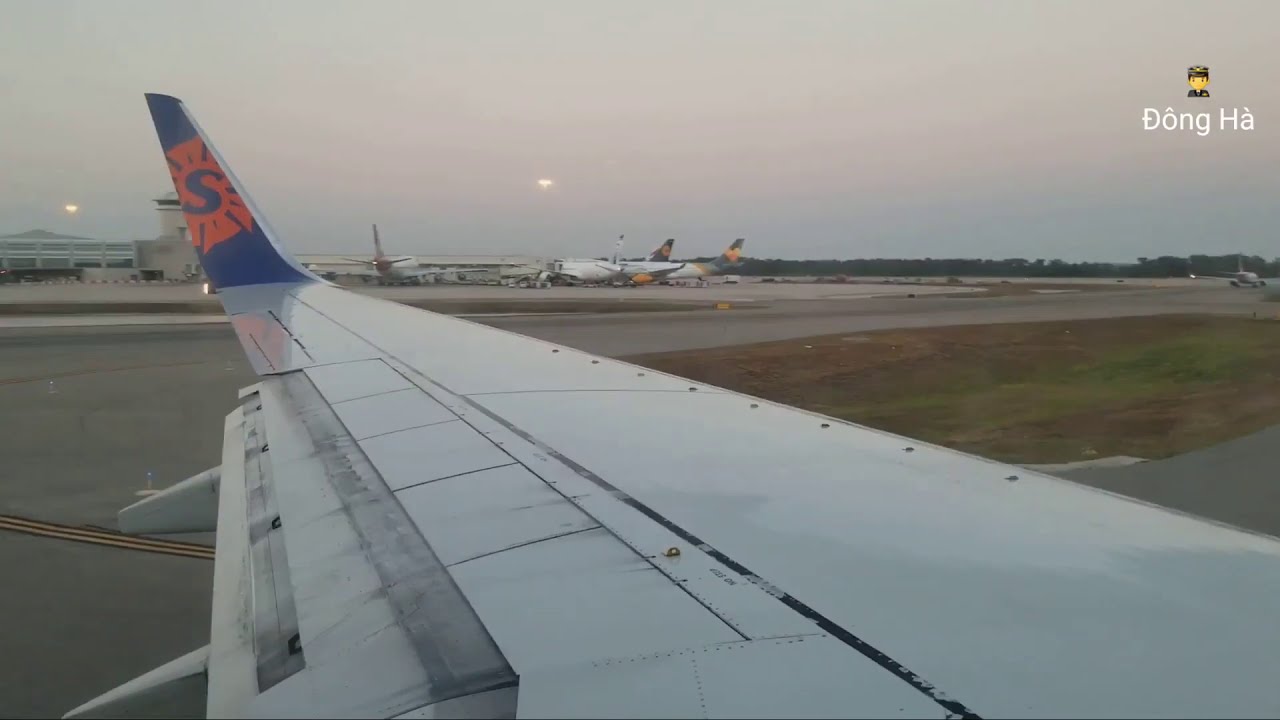This image captures the view from within a passenger jet, looking out over the wing towards an airport runway. The jet's long, white wing dominates the foreground, culminating in a folded wingtip displaying a blue and orange logo resembling a flower, with a blue "S" at its center. The scene appears to be at dawn, with a hazy, low light casting a soft pink and gray hue over the sky. In the background, several other aircraft can be seen on the runway amidst a mix of concrete and grassy surroundings. Towards the horizon, airport buildings and a line of trees are faintly visible. The overall color palette is composed of muted grays, blues, whites, and the occasional splash of orange, contributing to the serene yet bustling atmosphere of the airport prepping for early morning departures.